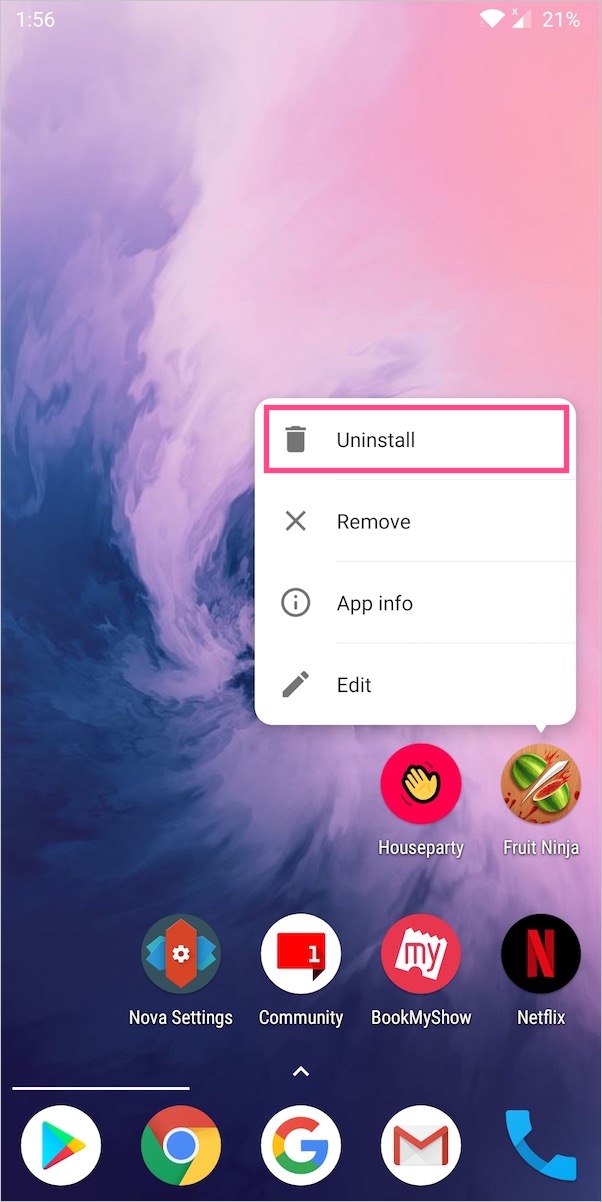This is a mobile device screenshot featuring a visually captivating home screen. The top of the screen displays an array of white status icons, including indicators for time, Wi-Fi connection, network connection, and battery status. At the bottom, shortcut icons provide easy access to essential applications such as the Google Play Store, Google Chrome Browser, Google Search, Gmail, and the phone app for making calls.

The background of the home screen is an ethereal cloud-like texture, blending dark blue, pink, and purple hues to create a mesmerizing, swirling smoke effect. Prominently displayed on the screen is a pop-up menu related to the Fruit Ninja application, offering four options: Uninstall, Remove, App Info, and Edit. The Uninstall option is distinctly highlighted with a pink rectangular box, indicating it is currently selected.

Beneath the pop-up menu, there are six additional app icons neatly arranged, completing the organized and visually appealing layout of the home screen.